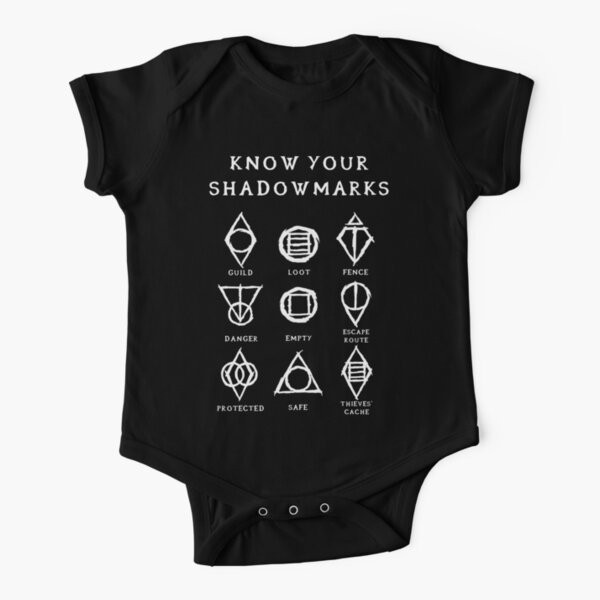The image depicts a black, short-sleeved baby onesie with a button fastener at the bottom, designed for infants. The onesie features white text and symbols on the front, with the bold text "KNOW YOUR SHADOW MARKS" at the top. Below this text are three rows, each containing three symbols accompanied by corresponding labels. The top row includes: "Guild" represented by a circle inscribed in a kite, "Loot" depicted as a rectangle with horizontal lines within a circle, and "Fence" shown as a diamond shape. The second row features: "Danger" as an upside-down triangle with a circle at the tip, "Empty" represented by a square inscribed in a circle, and "Escape Route" shown as a circle with a triangle at the bottom. The final row includes: "Protected" depicted as two intersecting circles with a diamond in the middle, "Safe" represented by a circle inside a triangle, and "Thieves' Cache" as a rectangle with horizontal lines within a kite. The background of the image is plain white.